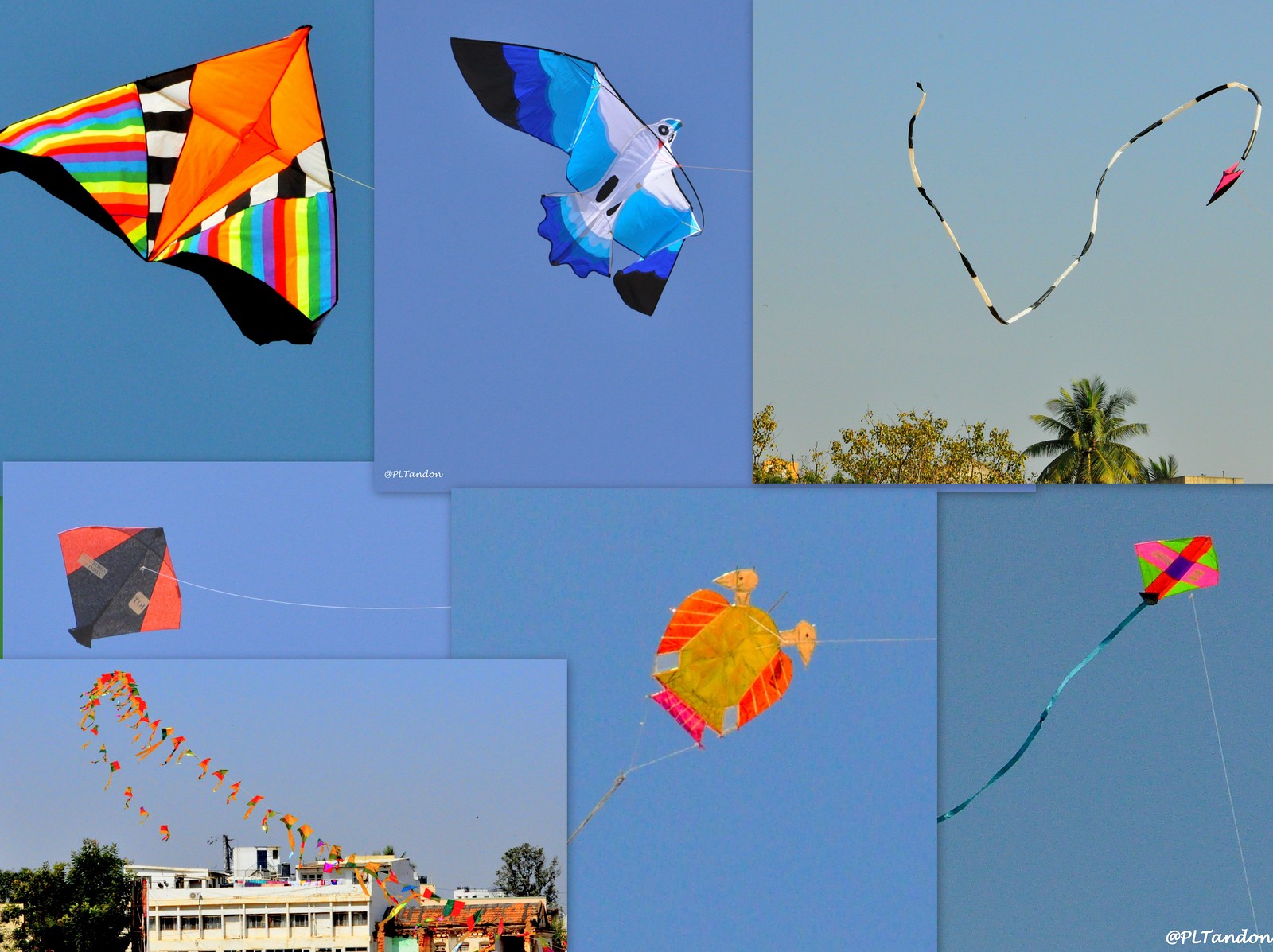This image is a horizontal rectangular collage composed of seven smaller photographs, all featuring kites against a backdrop of clear blue skies. In the top left corner, there is a striking triangular kite with vibrant orange, white, black, and rainbow-striped patterns on its wingtips. Next to it, in the center top position, a kite mimicking a blue bird showcases a beautiful gradient from light to dark blue, with black-tipped wings and a tail transitioning from white to dark blue. The top right image features a serpentine kite with a red head and a long tail patterned in black and white, looping gracefully like an 'S'.

On the center left, a square-shaped kite displays a bold black and red design. Adjacent to it, a whimsical yellow kite resembling a bug or crab has orange accents. The bottom row starts with an image in the lower left, showing a cluster of numerous vibrant kites and streamers fluttering together, creating a lively, colorful spectacle. Next to it, a kite with a green square body has a pink and red cross design and a black tail. The collage is artistically signed "PL Tandon" in white text in the bottom right corner. The bright sunlight emphasizes the vivid colors and dynamic shapes of the kites.